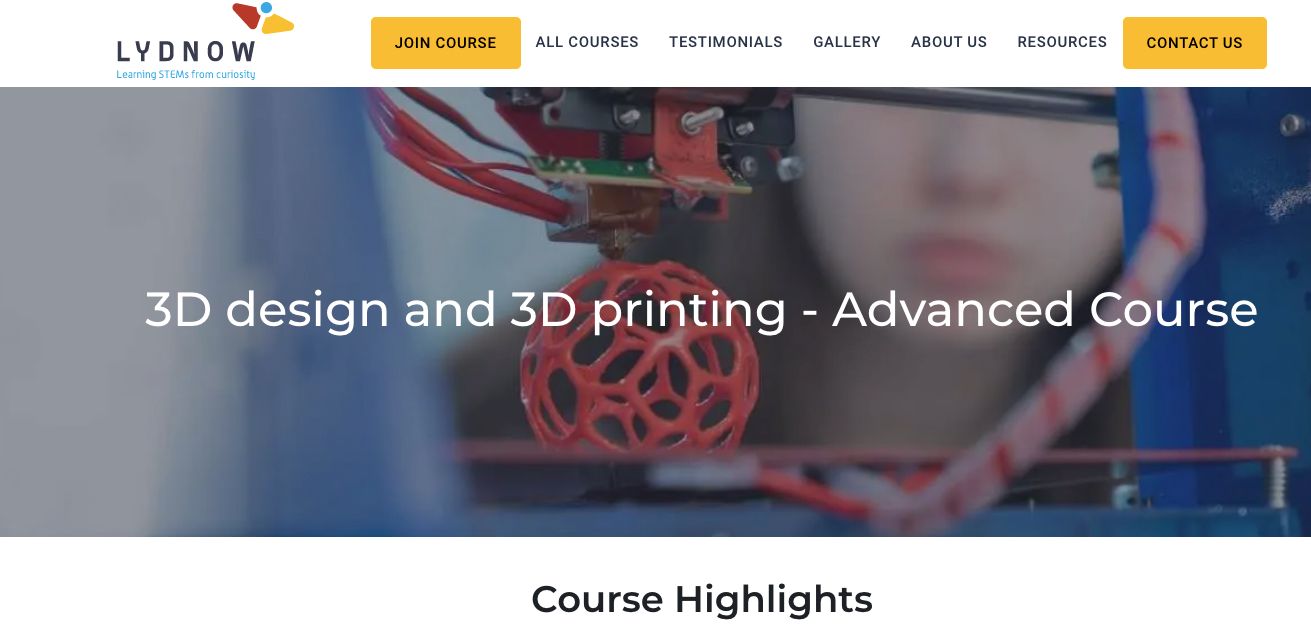The image appears to be a screenshot from a website, with "Lindau" prominently displayed in black text in the upper left corner. Adjacent to the title is a logo, which resembles either a bird or a plane, with vibrant red and yellow wings, and a small blue dot representing its head. Below the logo, the phrase "Learning stems from curiosity" is inscribed. 

To the right, a "Join Course" button is prominently highlighted by a large yellow rectangle. Surrounding this button are several clickable text options in black, including "All Courses," "Testimonials," "Gallery," "About Us," "Resources," and "Contact Us," with the latter also highlighted by a yellow rectangle.

Dominating the screen is a large rectangular image depicting advanced technology, specifically a 3D printer producing a red ball with a complex, web-like design. To the right of the printing process, a blurred image of a woman with fair skin and pink lips is faintly visible. Overlaying the image, white text reads: "3D Design and 3D Printing Advanced Course."

Beneath this image, in black text, the phrase "Course Highlights" offers further information about the course content.